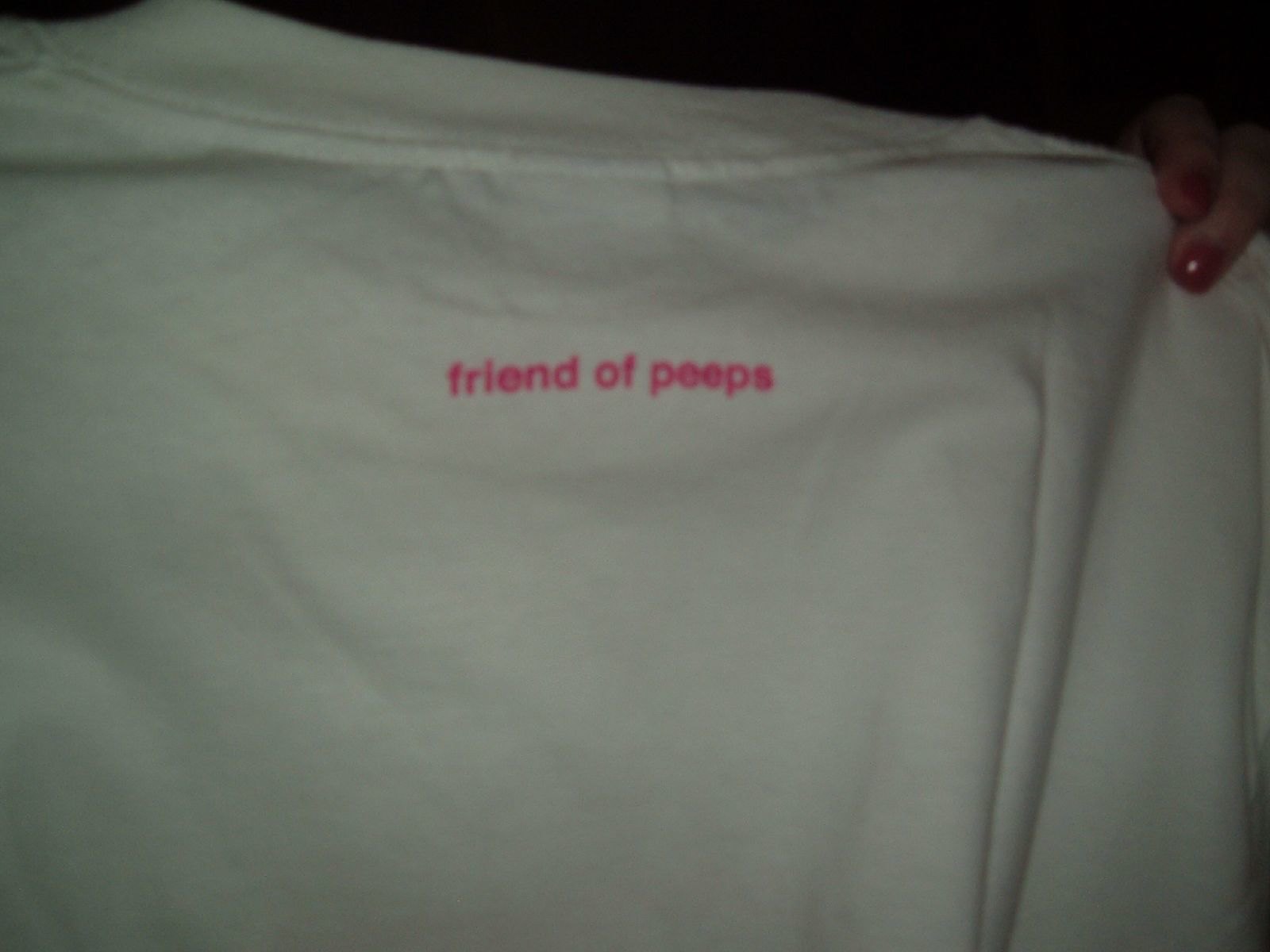In this dimly-lit photograph, a person with lighter skin tone is seen holding up a white t-shirt. The individual appears to be presenting the shirt to the camera, with only their thumb and index finger visible on the right-hand side, pinching the fabric. These fingers are adorned with shiny, deep red nail polish. The t-shirt features the text "friend of peeps" emblazoned in bright pink lowercase letters approximately two or three inches below the collar, which is positioned at the top center of the image. The background is entirely dark, highlighting the contrast between the t-shirt and its surroundings. The photograph captures subtle reflections on the fingernail polish, adding a touch of detail to the scene.